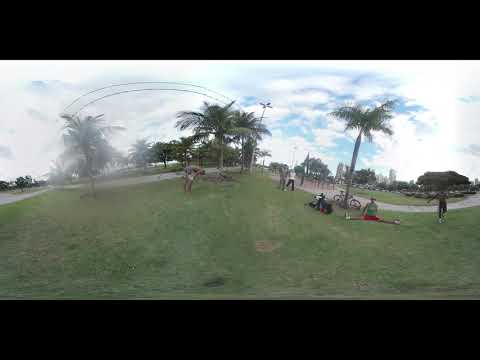This vertically rectangular image showcases a park scene filled with vivid details. Dominated by lush, flat green grass, the park features a sloping landscape that rises towards the center before descending towards the right. The sky above is a brilliant blue, dotted densely with white clouds, indicating a very cloudy yet bright day. 

A noticeable horizontal black stripe frames the top and bottom of the image, adding a unique visual effect. The overall image appears slightly warped, creating a wavy, distorted perspective. 

In the park, tall palm trees with long, swaying leaves are scattered throughout. One prominent tree on the right has several people gathered around it, with a bicycle rested against its trunk. Among the individuals, a person in a green tank top and red shorts is sitting on the grass with their legs spread wide. Not far from this scene, another person appears to be bent over, possibly injured, adding a dynamic human element to the setting. 

The park is crisscrossed by light gray concrete walkways, and in the distant background on the right, you can make out the dark brown rooftop of a small, one-story building. Further in the distance, tall buildings loom, providing a contrast to the natural, serene environment of the park. The combination of these detailed elements paints a comprehensive and bustling view of a typical day in this urban green space.